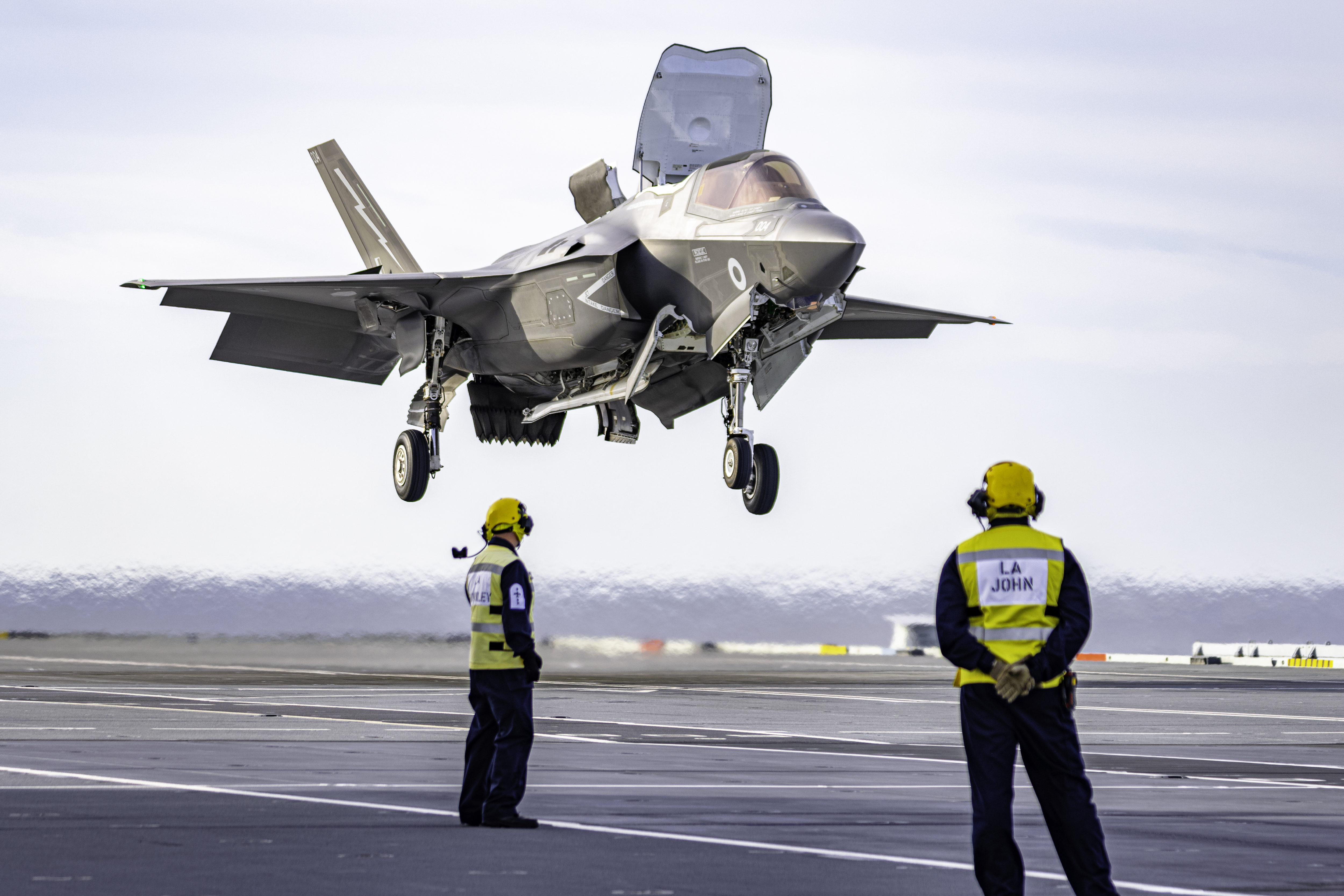In the photograph, we're at a military airbase, observing a dramatic scene. Dominating the image is a fighter jet, likely a vertical take-off type, hovering with its landing gear extended, clearly in the process of landing. The jet’s sleek, sharp nose resembles a bird's beak, and its air scoop is prominently visible at the front. The wings are equipped with lowered flaps, a closed canopy, and an open hatch at the top. Beneath the jet, the bay doors for the retractable wheels remain open, adding to the technical intricacy of the scene.

In the foreground stand two men, intently watching the jet. They are clad in dark uniforms—black pants and jackets—adorned with bright yellow vests and helmets for high visibility. They also wear heavy ear protectors, a necessary precaution in this noisy environment. Noteworthy is a sign on the back of the man to the right, reading "L.A. John." The background of the image features a light-colored sky, providing a stark contrast that highlights the jet and its spectators.